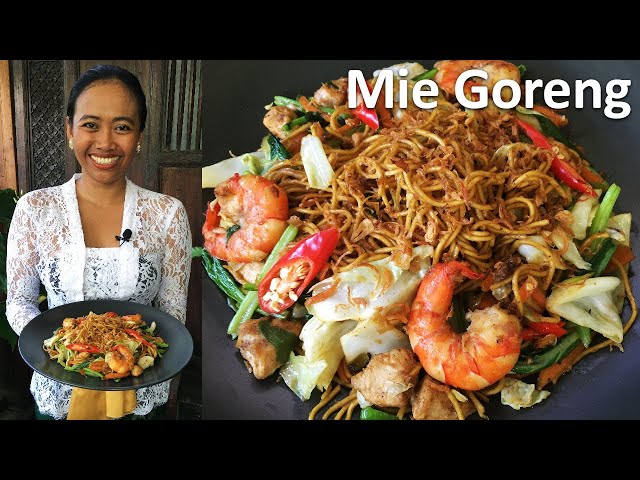This composite image features two side-by-side photographs against a black background. The photograph on the left showcases a smiling Asian woman with tan skin and pinned-back hair, wearing a lacy white blouse and earrings. She's holding a black plate of food in one hand. Behind her, a wooden wall or doorway can be seen. The photo on the right is a close-up of the dish she’s holding, named "MIE GORENG" as indicated by large white text at the top right of the image. The dish is a stir-fry of fried noodles adorned with shrimp, chili peppers, cabbage, and a variety of other vegetables.